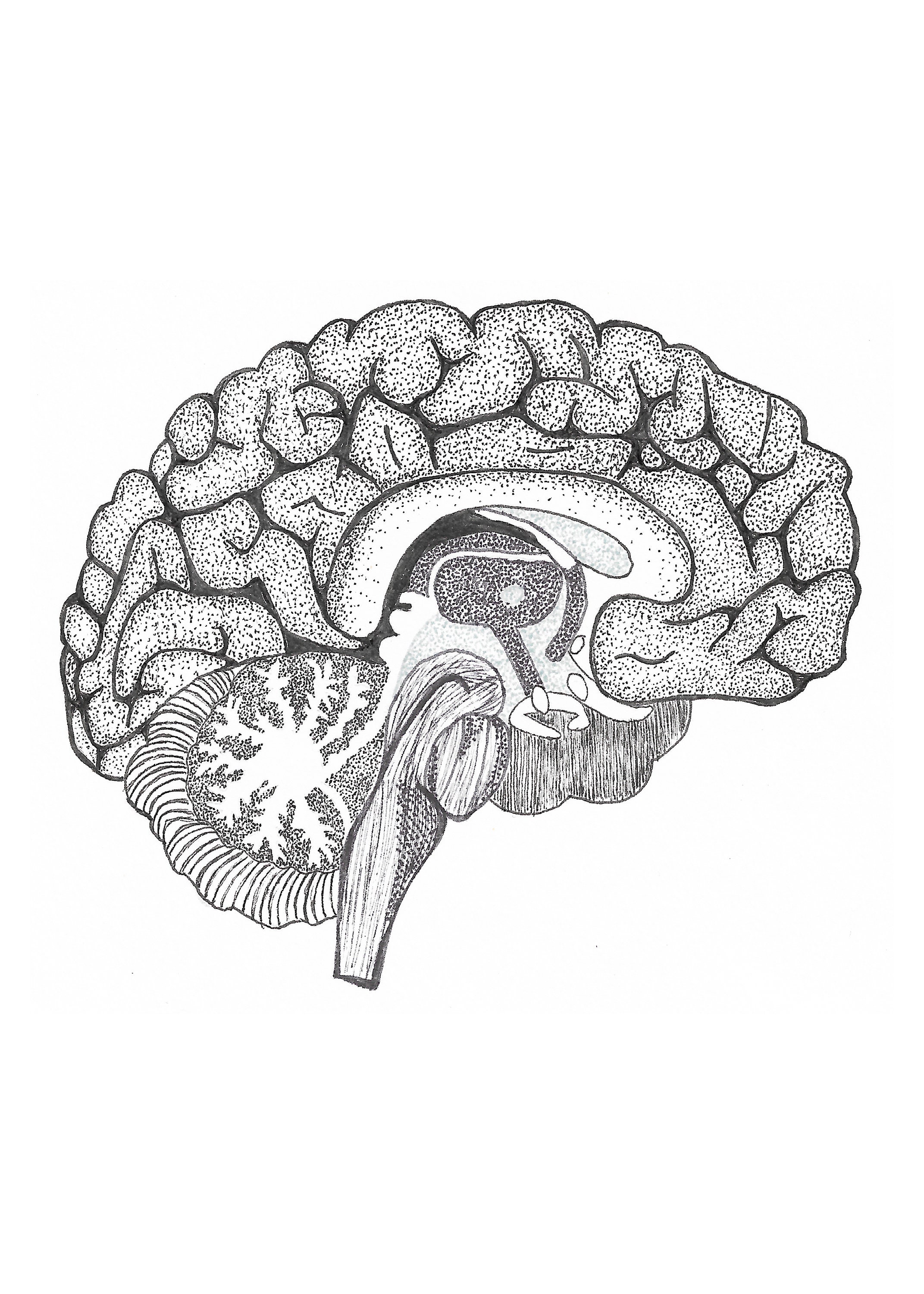The image is a detailed, black-and-white pencil drawing of a brain set against a completely white background, with no labels or annotations. The drawing shows one hemisphere of the brain viewed from the center, capturing intricate details of various brain structures. You can distinctly see the folds of the cortex adorned with small black pockmarks, adding texture to the drawing. The cerebellum and brain stem are also clearly visible, along with the corpus callosum. The shading techniques employed suggest the work of someone proficient in anatomical illustrations, possibly for use in a textbook or for studying anatomy. Although the purpose of the illustration isn't specified, the careful shading and level of detail imply it was created with an educational intent in mind.